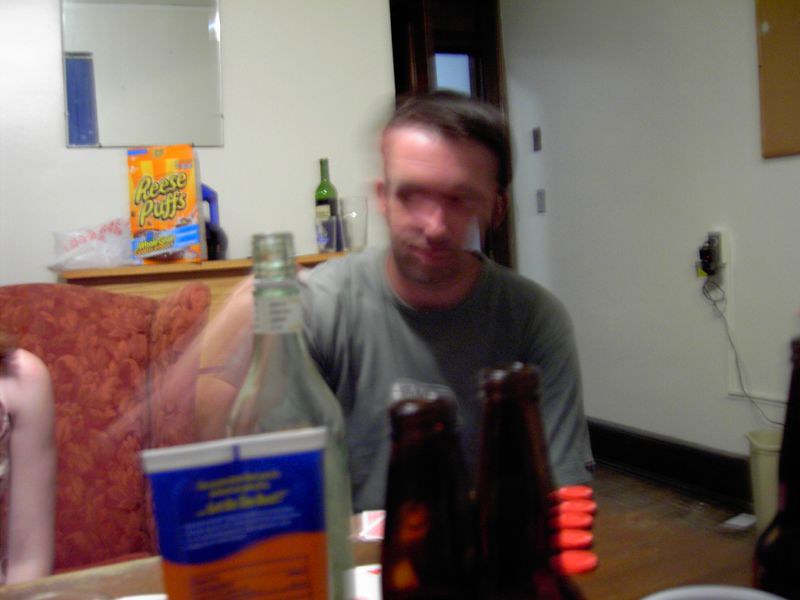This blurry indoor photograph appears to have been taken in a dimly lit room, possibly a kitchen or a work break room, with white walls and a somewhat cluttered atmosphere. The focal point is a man with straight black hair, parted to the left, and a short beard, dressed in a gray t-shirt. His face is indistinct due to the blurriness of the image, though he seems to be smiling slightly.

In the foreground, multiple bottles are visible on the table, including a couple of brown beer bottles and a clear glass bottle, possibly a wine bottle. There's also a small blue and orange container that might be holding sunscreen, as well as a bottle that resembles one used for ointment. Scattered among these items are cards and a row of red poker chips, suggesting a poker game might be taking place.

To the left of the man is an upholstered chair with a dark red fabric and lighter peachy-apricot designs, while a shelving unit or bureau stands behind him. On this unit, there is a vividly colored orange and yellow box of Reese's Puffs cereal, identifiable by its distinctive yellow print. Beside the cereal box, there appears to be another wine bottle, a green glass bottle of red wine, accompanied by a couple of glasses. A door is partially visible in the upper center of the photo, and a mirror hangs on the wall to the upper left.